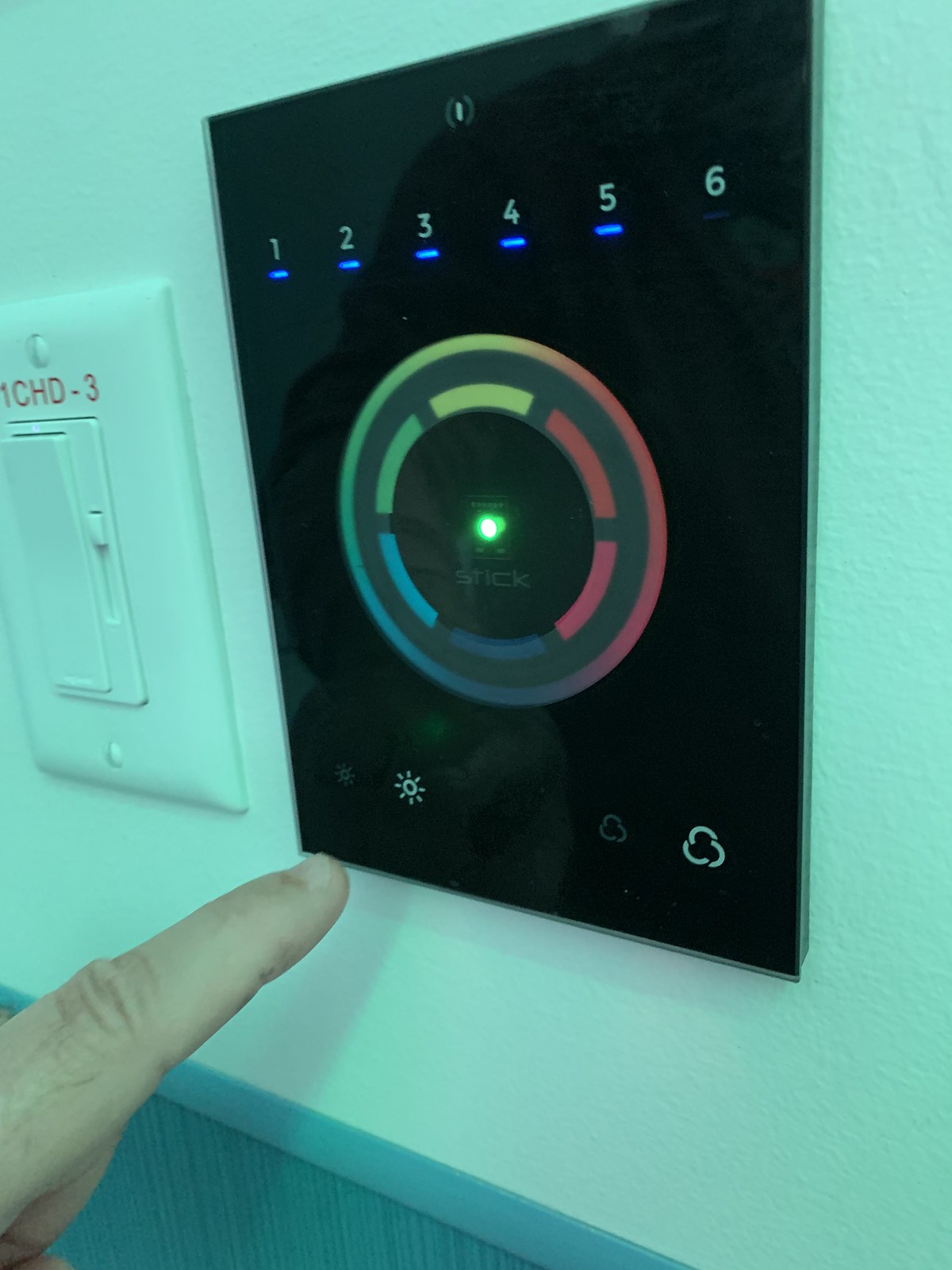The photograph captures an individual standing in front of an array of control panels mounted on a white wall with distinctive wainscoting. The wall showcases a combination of design elements: the lower half features bluish striped wallpaper separated from the white upper half by a wooden trim in a lighter blue hue. The painted portion of the upper wall appears to be cement with a slightly lumpy texture.

On the left side of the image, the person's left index finger points towards a black panel, possibly made of glass or plastic, reflecting parts of the person's shirt and arm up to the shoulder and chest area. To the left of this panel, a white levered switch for a light is visible. This switch teeters back and forth and features the label "1CHD-3" at the top, alongside a dimmer slide bar on its right side.

The black panel itself has various elements. At the top, within brackets, there is the number "1," followed horizontally by six numbers, each with a blue indicator light below it. The first five blue lights are illuminated, while the last one remains dark. Along the bottom of the panel are buttons for adjusting brightness, with the individual seemingly aiming to increase it. 

The central area of the black panel prominently displays the logo "STICK." Just below the logo, a very bright green light emanates from the center of a circular color wheel. This central circle, segmented into six equal parts, displays colors in the following order clockwise: yellow, green, light blue, purple, reddish, and orange. Surrounding this segmented circle is a thinner outer circle with a gradient blend of the same colors, creating a continuous color spectrum.

The precise function of the interface remains unclear, but it appears to be a sophisticated control panel likely used for adjusting lighting or other environmental settings.